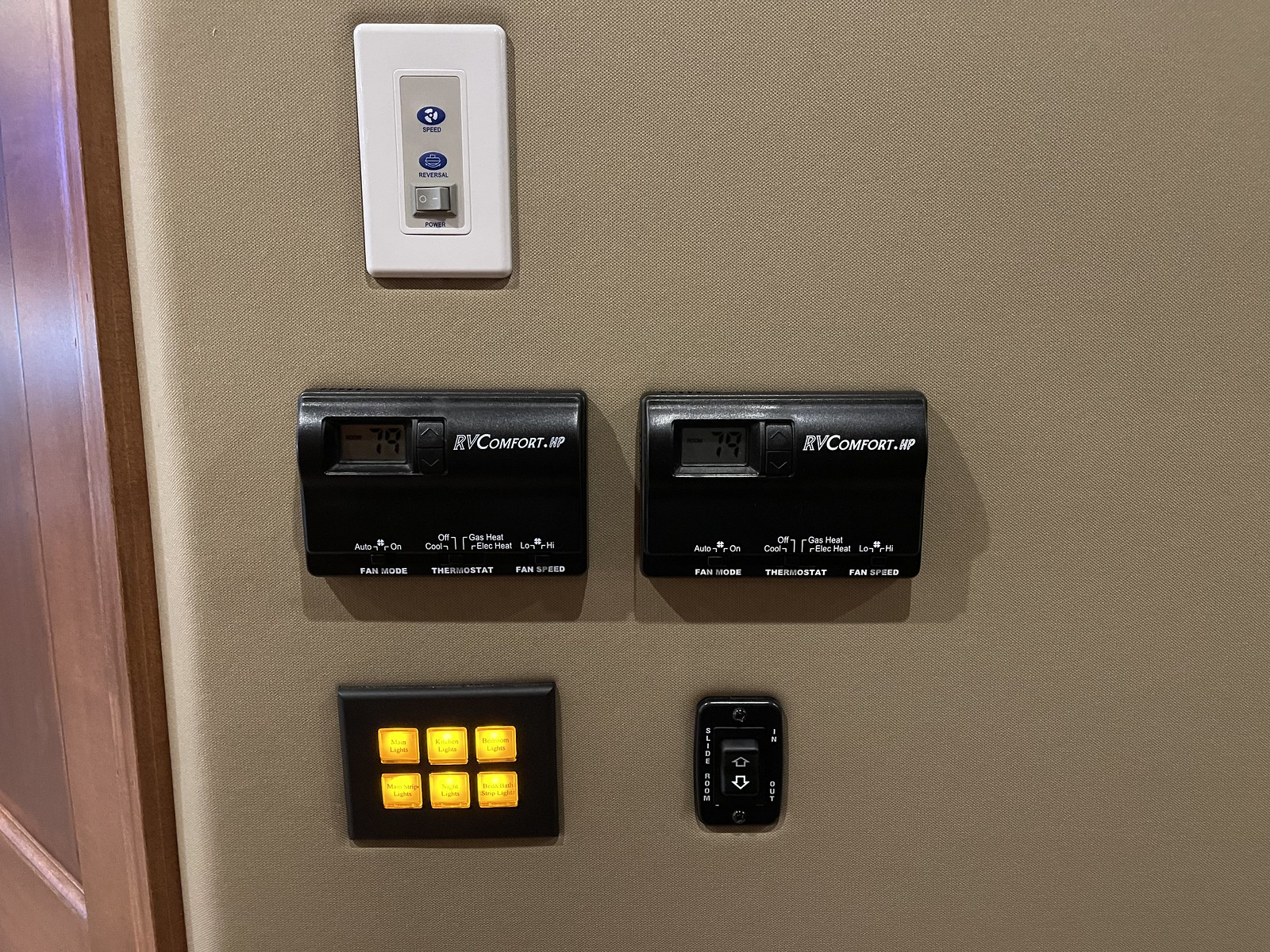The photograph captures a section of a recreational vehicle's interior wall that is outfitted with various climate control and outlet features. The focal point is a tan fabric-covered corner, transitioning to a wood-paneled section. Mounted at the top of the wall is a white bracket, which appears to be a fan switch. This switch features a blue circle indicating fan speed and another blue circle with an icon for reversal, alongside a gray switch labeled "Power." Below this setup are two black control units marked "RVComfort.HP," both displaying a readout of 79°F. These units offer a range of settings, including "Auto," "Cool Off," "Gas Heat," "Electric Heat," "Fan Mode," "Thermostat," and "Fan Speed." Lastly, a black control panel with six illuminated yellow buttons is situated lower on the wall, designed to manage the RV's lighting.